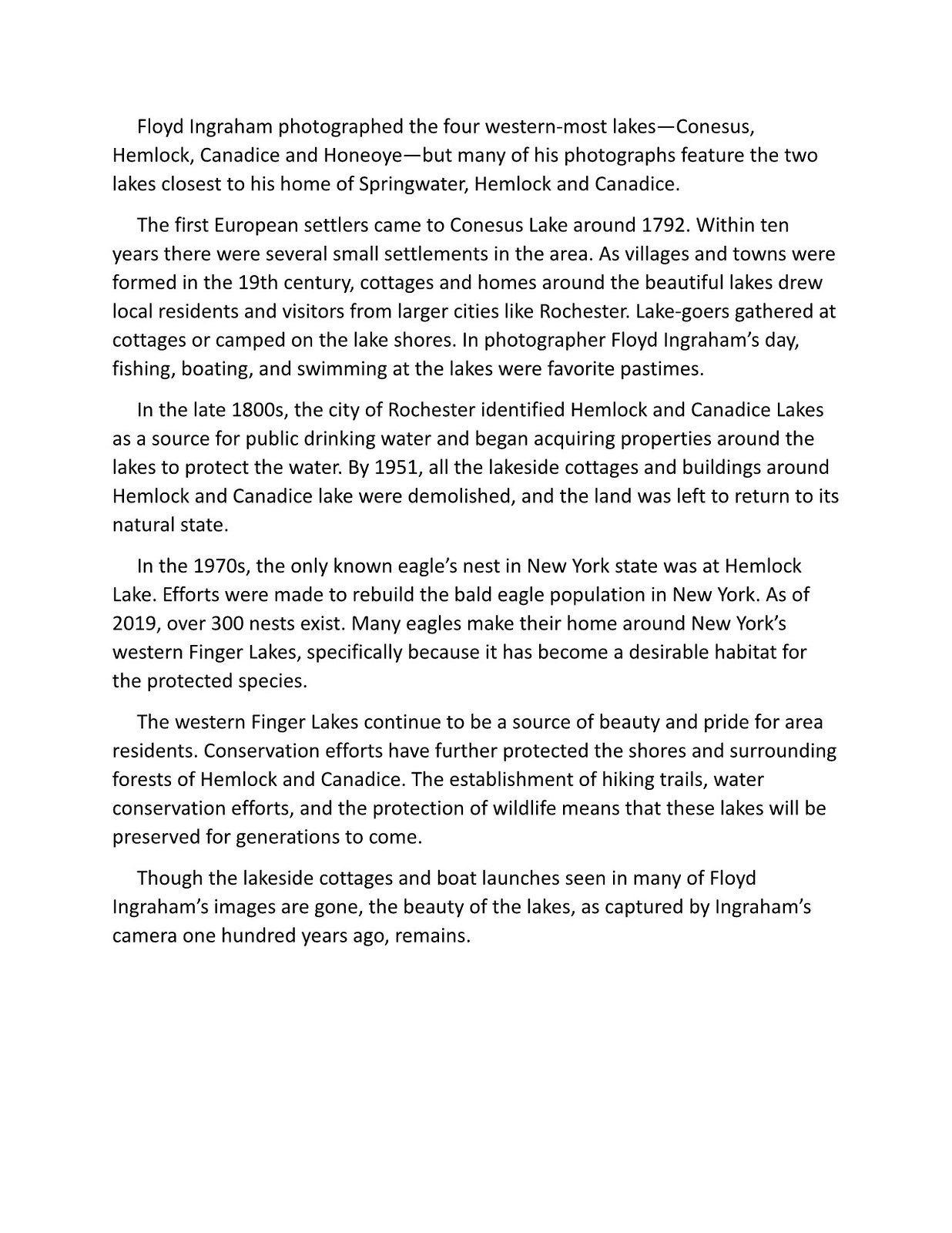This image appears to be a page from a book or an article, set against a white background with black text, detailing the history and photography of the Western Finger Lakes in New York by Floyd Ingraham. Floyd Ingraham is known for photographing the four westernmost lakes—Conesus, Hemlock, Canadice, and Honeoye. Most of his collections prominently feature Hemlock and Canadice, the two lakes closest to his Springwater home. The narrative mentions that Conesus Lake saw its first European settlers around 1792, with small settlements growing within ten years. By the 19th century, the picturesque lakes attracted local residents and visitors from larger cities like Rochester, who enjoyed fishing, boating, and swimming. In the late 1800s, Rochester identified Hemlock and Canadice as public drinking water sources, leading to property acquisition around these lakes and the eventual demolition of lakeside cottages and buildings by 1951 to protect the water quality. The 1970s saw New York's only known eagle's nest at Hemlock Lake, sparking efforts to restore the bald eagle population, which expanded to over 300 nests by 2019. These lakes, part of New York's Western Finger Lakes, are now cherished for their natural beauty and conservation efforts, which include hiking trails and wildlife protection. While the lakeside cottages and boat launches from Ingraham’s era are gone, his photographs continue to immortalize their enduring beauty.